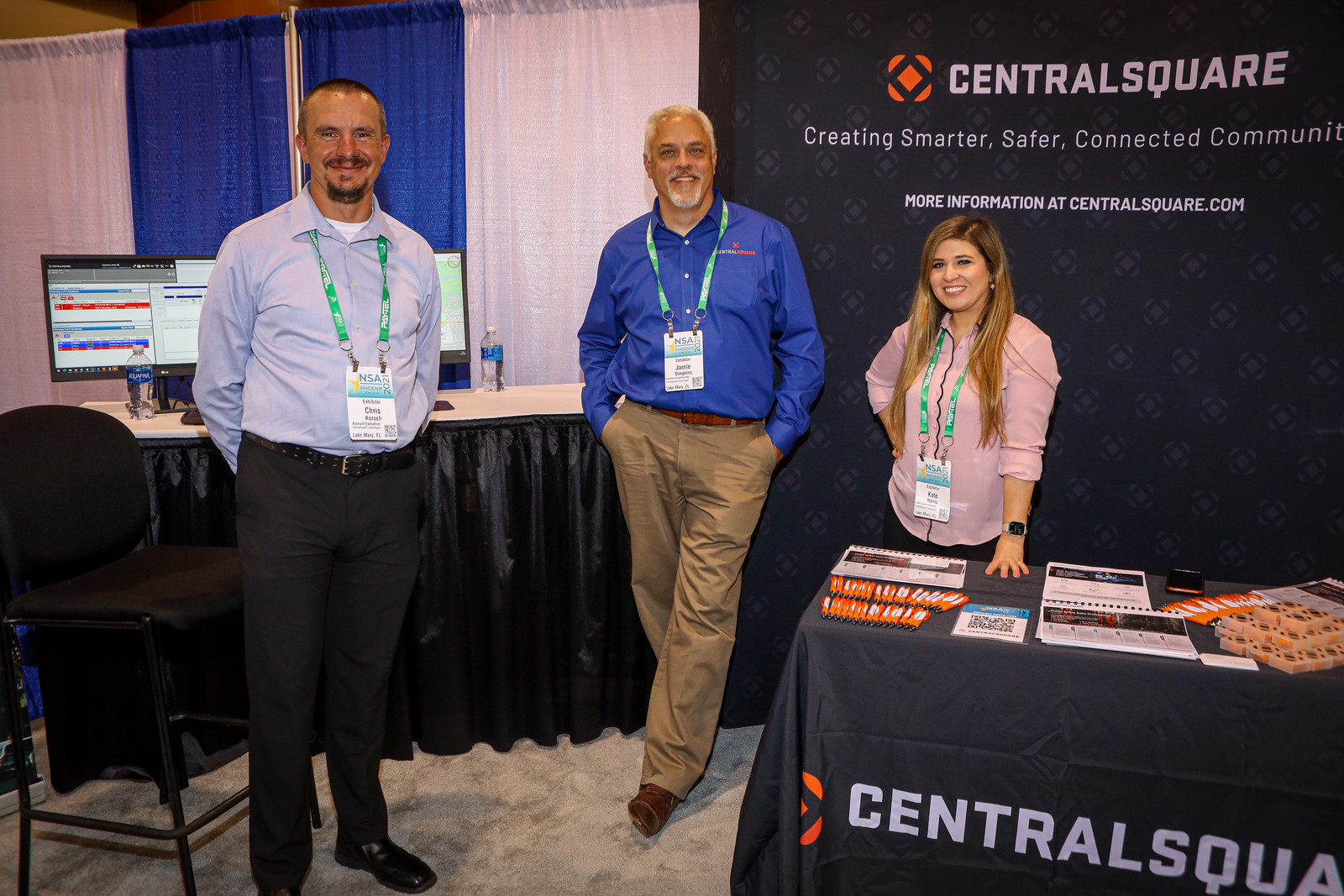The image features three individuals – two men and one woman – standing behind a table draped with a black tablecloth bearing the "Central Square" logo, an orange square, and the slogan "Creating Smarter, Safer, Connected Communities." A black banner behind them reiterates this slogan and provides more information at centralsquare.com. 

The man on the left is wearing a green lanyard with "NSA Phoenix" and his name tag attached, a gray collared shirt, and black khaki pants. He has short hair. The man in the middle is dressed in a light blue long-sleeved shirt and brown khaki pants. He sports gray hair and a gray goatee and looks cheerful. The woman on the right has long blondish-brown hair and is wearing a pink long-sleeved button-up shirt with the sleeves rolled up and black pants. A pair of computers and water bottles are visible on a table behind them, with a black curtain hanging below. The table in front of them is adorned with calendars, assorted literature, and orange pens. 

The overall setup suggests the trio is prepared to present or showcase information about Central Square, emphasizing a professional and organized atmosphere.